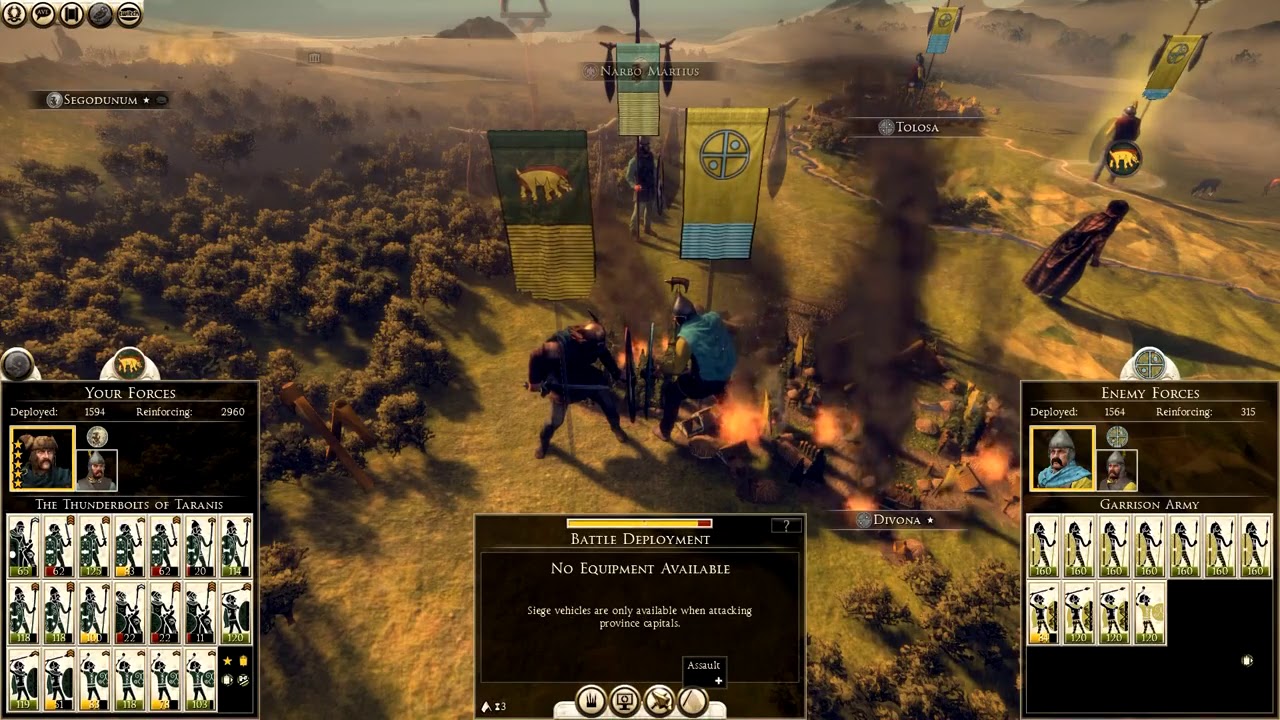The image is a detailed screenshot from a medieval-themed strategy video game, capturing an outdoor scene on a flat landscape with rolling hills. The camera angle is an aerial view, focusing on an open battlefield divided by a dense forest on the left and a grassy clearing on the right. Central to the scene are two towering characters in medieval knight armor, vastly oversized compared to the surrounding environment, and they are facing each other. Each knight holds large standing banners—one is adorned with gold, blue lines, and a circle with a cross and dots, while another features a warthog emblem.

The interface displays vital game information. On the lower left, a black box titled "Your Forces" shows the player's available soldiers and their status, along with images of key characters and unit cards arranged in rows. The bottom center of the screen prominently features a "Battle Deployment" label, indicating "No Equipment Available." On the lower right side, another black box titled "Enemy Forces" provides similar information about the opposing army, including their leader and army formation. Additionally, the backdrop reveals a small village with some structures catching fire, adding to the chaotic ambiance of the battlefield.